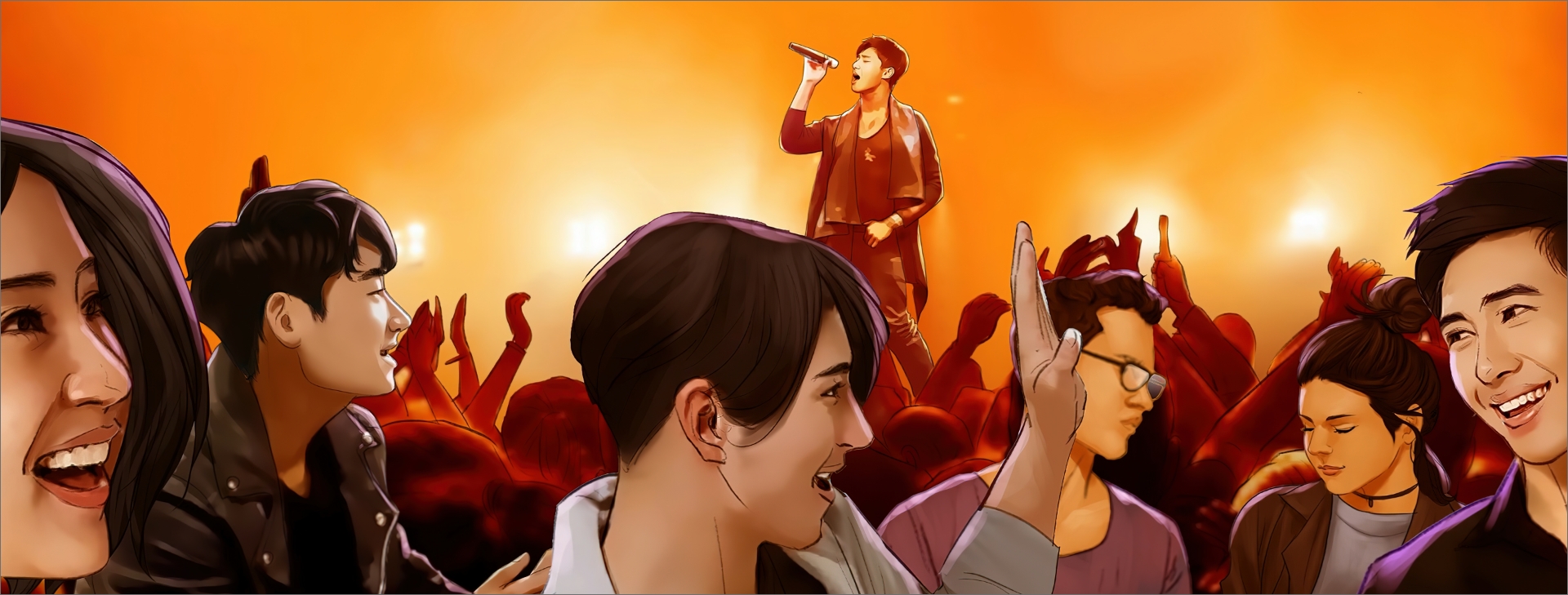The horizontally aligned rectangular image is an animated scene capturing the lively atmosphere of a concert. In the background, a young man with short dark hair stands on a stage, singing into a microphone. He is dressed in a brown outfit, complete with a long-sleeve shirt, pants, and a scarf around his neck, and faces towards the left side of the image. The stage is bathed in colorful blends of light orange and dark orange hues, punctuated by several white spotlights that add to the vibrant atmosphere.

In the foreground, a joyful crowd enhances the energetic setting. Among them, a man at the center raises his hand, seemingly about to give a high five to another man smiling broadly at him from the right side of the image. To the left, part of a woman's face is visible; she has long hair cascading down and is beaming widely, showing her teeth. The animated people in the crowd, some with brown hair, are engaged in dancing, laughing, and talking, adding to the festive mood. The interplay of warm background lighting and the enthusiastic audience creates a fun, energizing, and celebratory environment.